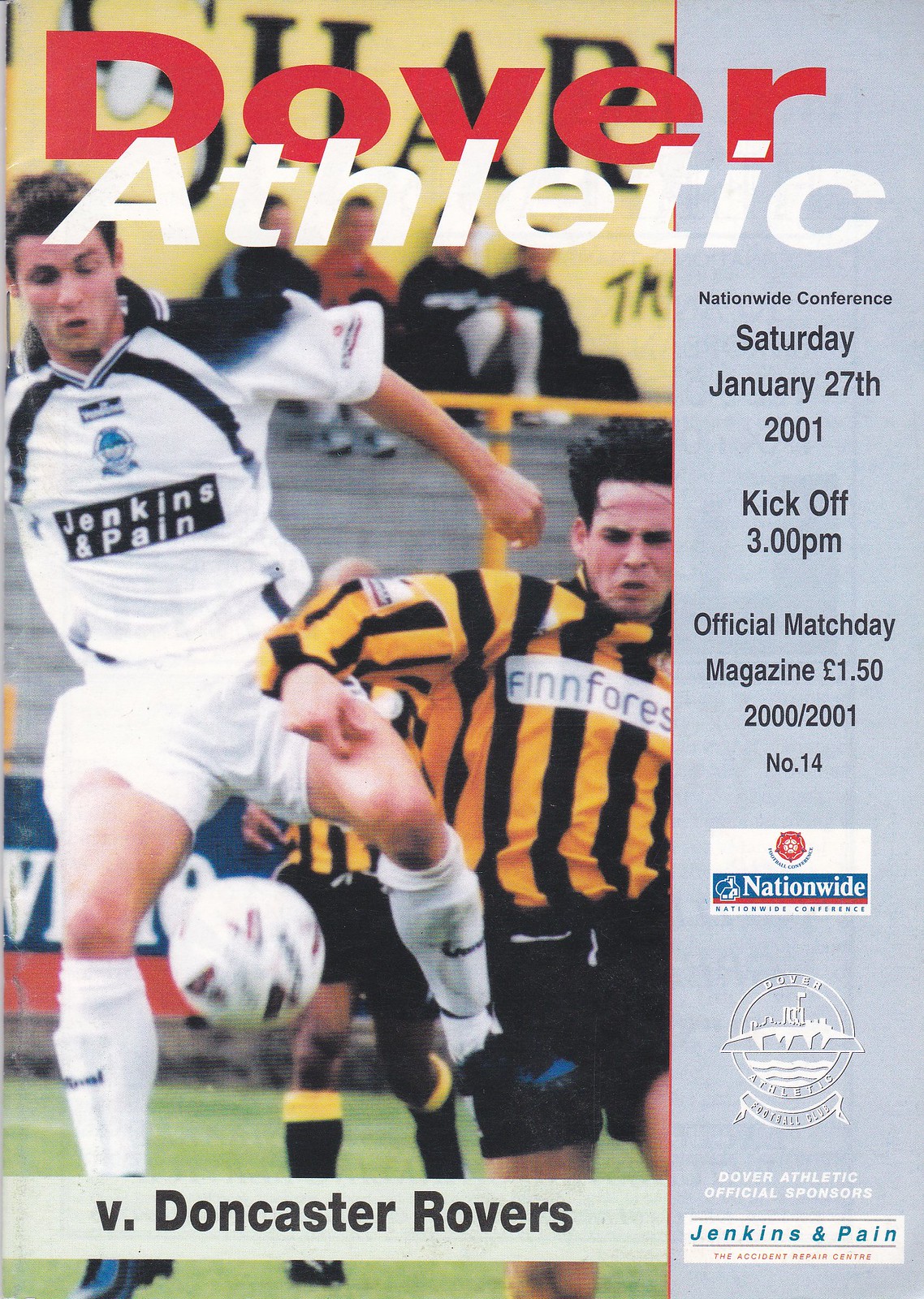The image depicts the cover of an official matchday magazine for Dover Athletic. The title "Dover" is prominently displayed in red font, with "Athletic" in white font across the top. At the center of the cover, a dynamic action shot features a soccer player in a white uniform with black stripes labeled "Jenkins and Payne" leaping into the air to kick a soccer ball. This player is oriented towards the viewer and positioned slightly to the left and in front of another player wearing a vertically striped yellow and black jersey with black shorts. A third player, also in a yellow and black striped uniform, appears in the background. 

The lower portion of the cover includes a semi-transparent banner stating "vs Doncaster Rovers". On the right-hand side, a light gray vertical section details additional information about the match: "Nationwide Conference, Saturday, January 27, 2001, kickoff 3 p.m, official matchday magazine, $1.50, 2000-2001, Number 14". This section also features the logo of Nationwide as a sponsor and additional sponsors including Jenkins and Payne Accident Repair Center.